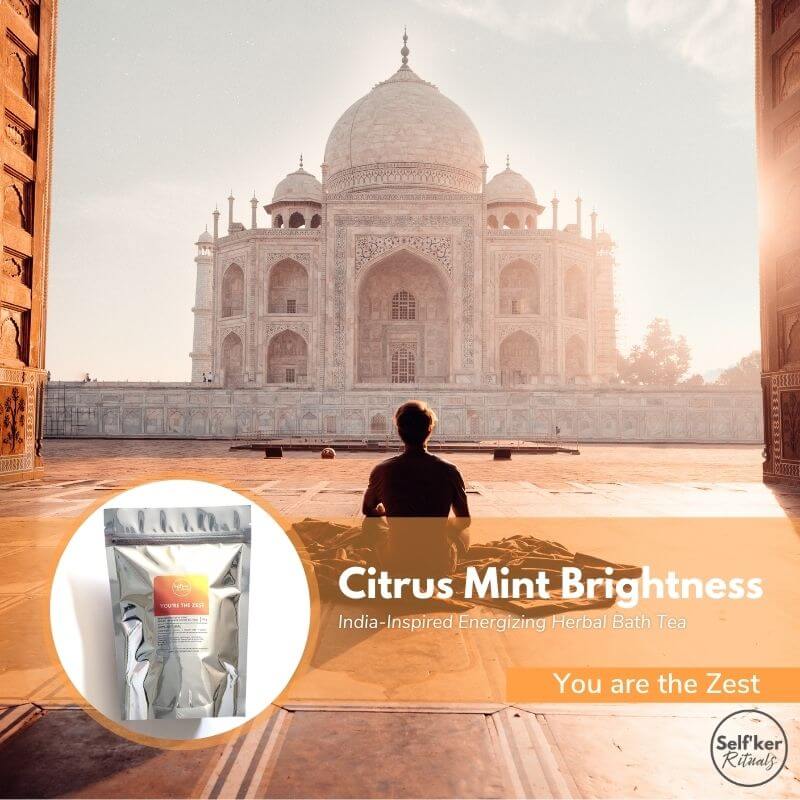In this advertisement for Citrus Mint Brightness, an India-inspired, energizing herbal bath tea, the scene is artfully composed. The background features a grand, ornate architectural building styled after Indian design, with a large central dome flanked by two smaller domes, framed by two-story arches that house big doors and windows. The building appears on a sandy beige backdrop, transitioning to white. 

In the immediate foreground, large floor tiles lead to a man seated on a blanket or towel, with his back to the camera, gazing at the architectural marvel ahead. Above the central section, white text on a warm amber, sandy-yellow background reads: "Citrus Mint Brightness" followed by "India-inspired energizing herbal bath tea," and a motivational line, "You are the zest," in darker mustard-colored text.

Adjacent to this text, on the left of the yellow banner, is a circular white area displaying the product—a silver and white package with a yellow and orange label. Additionally, a small logo at the bottom right corner, within a black circle, reads "self'KER rituals."

Overall, this detailed and visually appealing scene underscores the luxurious and invigorating nature of the advertised herbal bath tea.